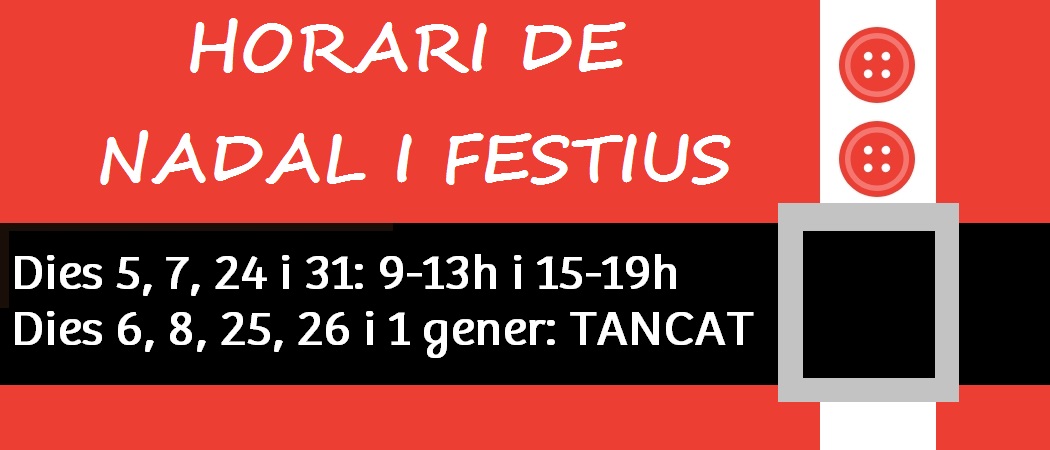The image features a festive, Christmas-themed banner with a light red background. At the very top, white text reads "Horary de Nadal I Festius." To the right, there's a vertical white rectangle with two red buttons and a silver belt buckle below them, evoking the appearance of a Santa suit. Centrally positioned, a black rectangular area (mimicking a belt) connects to the silver buckle, with white text detailing event dates and times: "Dyes 5, 7, 24 I 31: 9 to 13H, I15 to 19H." Below that, additional dates are listed: "Dyes 6, 8, 25, 26, I1 Janair: TANCAT." The overall design, dominated by red, white, black, and gray tones, invites viewers to a Christmas event, blending festive elements with crucial scheduling information.